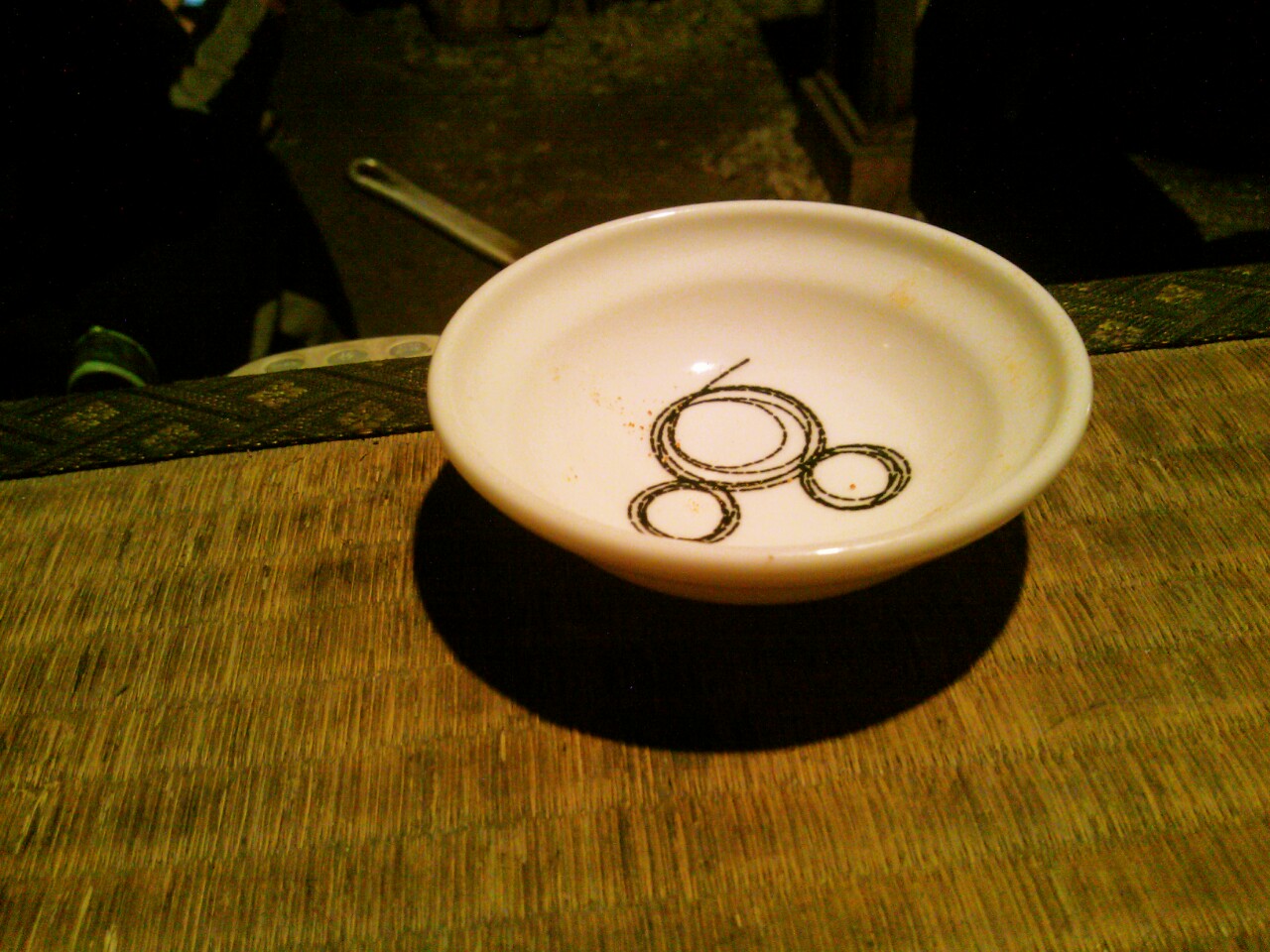This photograph captures a dimly lit kitchen scene centering on a cream-colored porcelain bowl adorned with a unique design resembling an outline of Mickey Mouse's head. This design features a large circle with multiple intersecting smaller circles, flanked by two smaller circles positioned like ears, each also containing intersecting circles, giving the appearance of intricately tangled yarn. The interior of the bowl is marked with orange and red stains, implying recent use. The bowl is situated on a brown and light brown tatami-lined table, characterized by tightly woven reeds and accented with a chocolate brown hue, along with embedded pink and green floral patterns set within diamond shapes formed by black and light brown lines. In the background, a silver pot handle is visible, emerging from a lower shelf, suggesting kitchen activity. Despite the dim lighting and some visible dirt on the floor, the focus remains on the detailed design of the bowl, which rests prominently within its intricate surrounding backdrop.